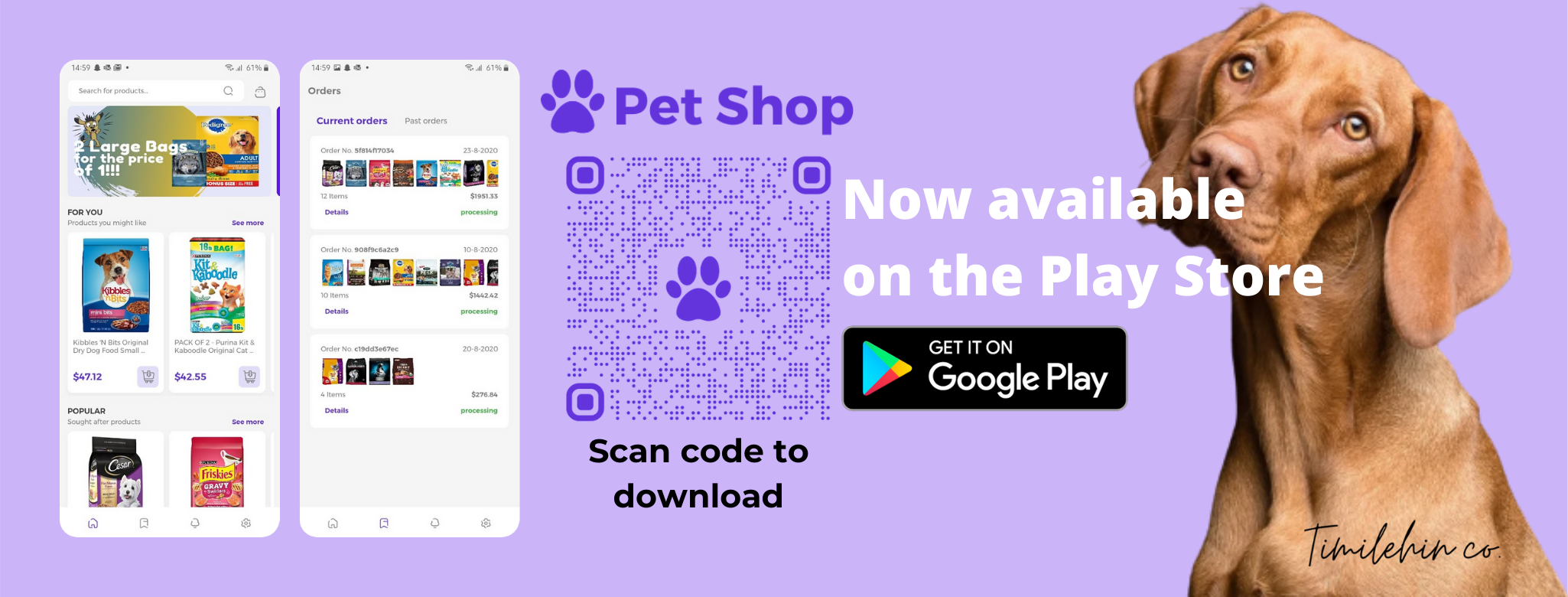The image appears to be an advertisement for a pet-related mobile application, likely focusing on online pet shopping or a pet game. The background features a horizontally oriented purple rectangle. 

On the right side, there's a picture of a medium-sized, short-haired brown dog with floppy ears, gazing sadly at the camera. 

The left portion of the image displays two smartphone screens. One screen shows various pet items, predominantly different types of dog food like Kibbles 'n Bits, Kit 'n Kaboodle, Friskies, and Caesar, along with a promotional text reading, "Two large bags for the price of one." The other screen illustrates a "Current Orders" section, listing different dog foods along with their prices and an indication that the order is "Processing."

In the center-right area of the image, there is a purple paw print logo accompanied by the text "Pet Shop." Nearby, a QR code is presented with a brief instruction to "Scan code to download," indicating the app is available on the Google Play Store with the message "Now available on the Play Store. Get it on Google Play."

The advertisement seems to be promoting a new mobile application related to pet shopping, emphasizing its convenience and special offers.